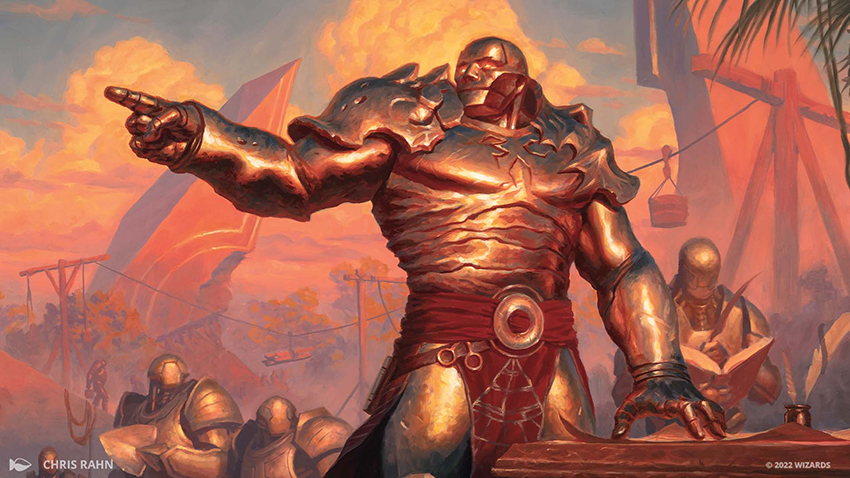The digital artwork, titled "Chris Rahn, 2022 Wizards," depicts a colossal, muscular warrior donned in iron-colored, gold-tinted armor with formidable shoulder pads and chest protection. The warrior, bald and emitting an aura of power with glowing red eyes, commands attention in this animated, landscape-mode piece. He points with his right arm, which is armored and lifted, while his left hand presses down on a piece of paper positioned on a table. A red cloth, secured with a silver buckle, drapes from his waist, covering his groin area.

In the immediate background, another armored figure is engrossed in writing with a quill in a book. To the left, two additional soldiers are visible, one with a spiked hand looming menacingly. The scene is set against a dark, orange-copper and blue sky, suggesting dusk or an impending sunset. This dramatic backdrop includes clouds, towering stone obelisks with intricate glyphs, wooden crosses bearing logs, and a distant green palm tree in the top right corner. The overall tone is gothic and intense, accentuated by the inscription of Chris Rahn in the bottom left corner and the year 2022 Wizards on the bottom right.